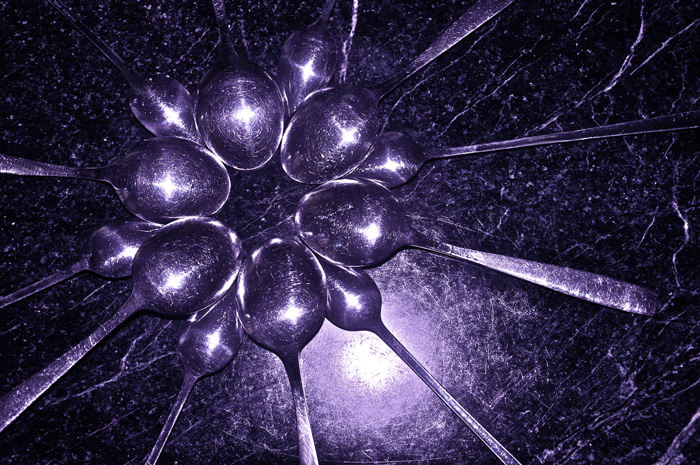The image captures an intricate arrangement of silver spoons on a black countertop, subtly veined with white. Illuminated by a light source above, the scene is striking with its interplay of light and shadow. At the center-left, twelve spoons are meticulously organized into a circular starburst pattern. This formation consists of six larger spoons, likely serving spoons, positioned upside down with their handles radiating outwards. Alternating between each larger spoon are six smaller spoons, possibly long-handled ice teaspoons, also placed upside down, creating a secondary ray of extensions. The reflection of the light source is vividly captured across the polished surface of the spoons, enhancing the visual effect. The black countertop, resembling either formica or granite, with its reflective quality and random spots, adds depth and contrast to the composition, making the spoon arrangement resemble a radiant sunburst.